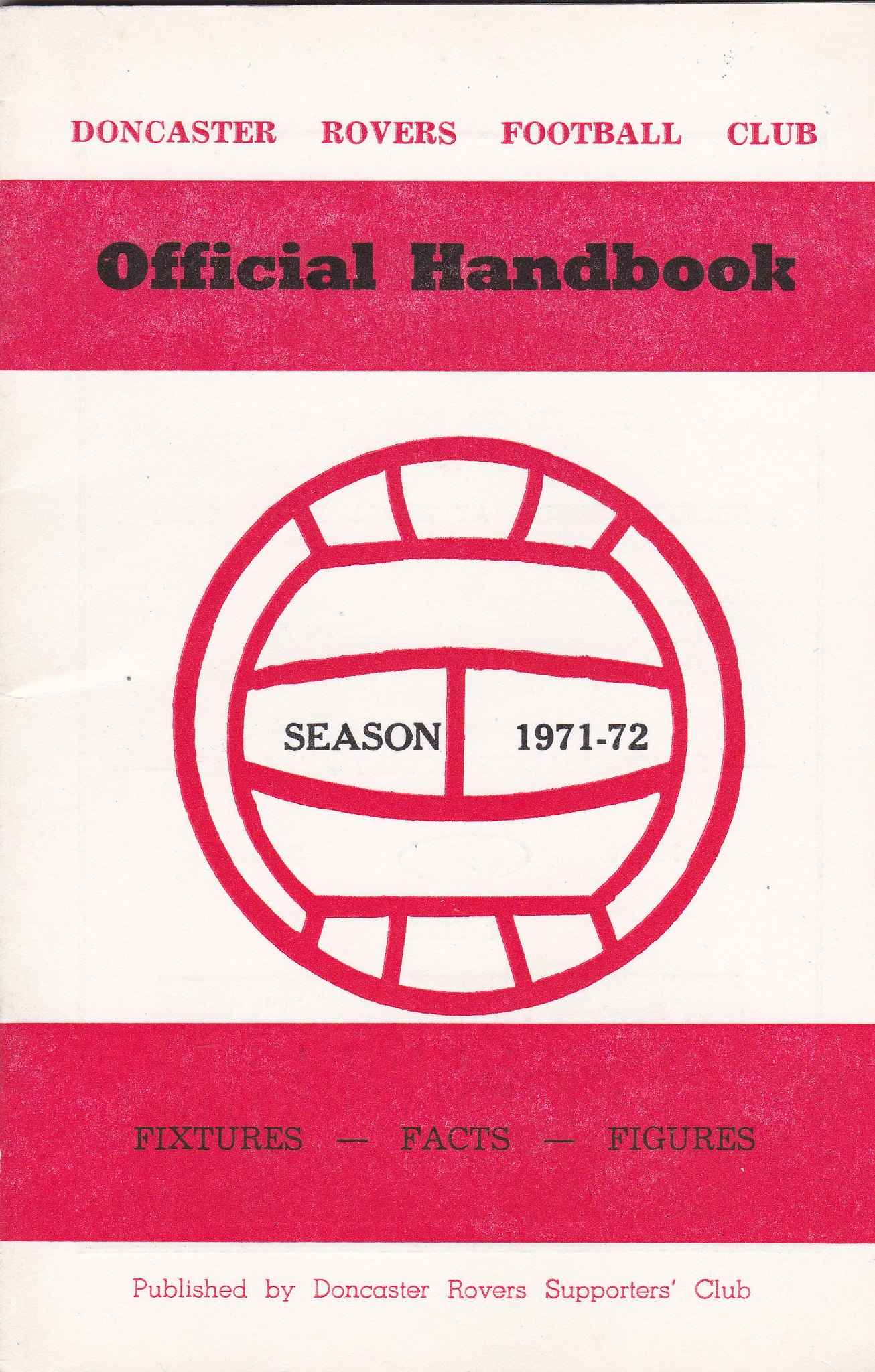The image depicts the cover of an official handbook for the Doncaster Rovers Football Club, likely for the 1971-72 season. The cover features a clean white background with prominent hot pink framing. 

Across the top is a red band containing the title "Doncaster Rovers Football Club" in white text. Below this, a hot pink band displays the text "Official Handbook" in black lettering. The center of the cover is dominated by a graphic of a white soccer ball, outlined in red, with black text inside it reading "Season 1971-72."

Underneath the soccer ball is another hot pink band with black text that states "Fixtures-Facts-Figures." The bottom of the cover returns to the white background with small red text reading "Published by Doncaster Rovers Supporters Club." This repetitive framing and consistent color scheme present a meticulously organized design, showcasing key information about the handbook effectively.